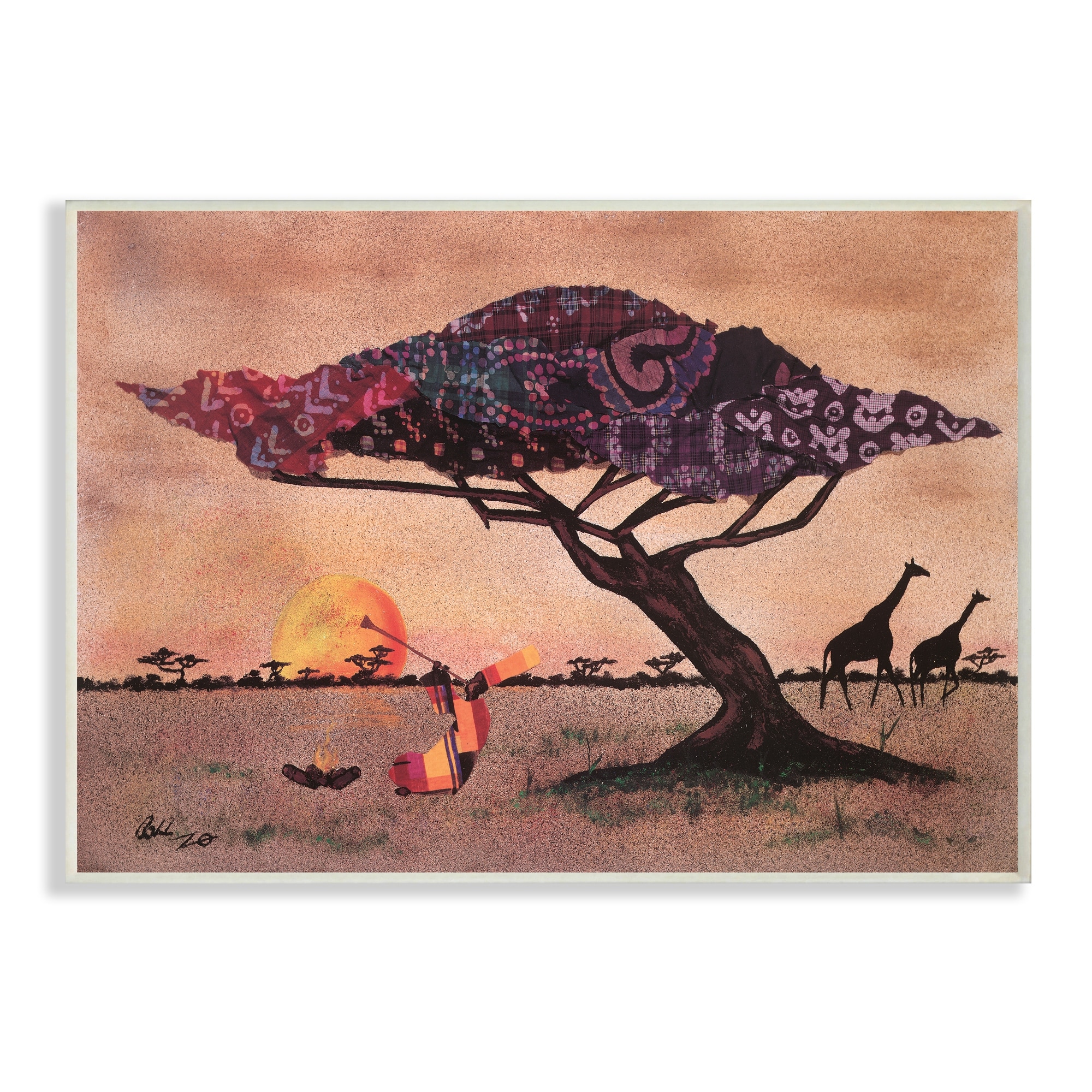This image is an artistic painting that vividly captures an African landscape. Central to the scene is a large, iconic tree with a dark brown trunk that leans to the left, spreading its wide branches horizontally. The foliage is uniquely adorned with intricate patterns in reds, purples, and greens, reminiscent of traditional African textiles used in women's clothing. Beneath this tree, an African man dressed in vibrant, striped attire—featuring shades of red, yellow, and orange—sits quietly by a burning campfire. He wears a long, similarly colored hat and appears to be playing a musical instrument. In the background, a sun sets dramatically on the horizon, casting a warm glow over the scene and silhouetting two giraffes on the right side. The landscape stretches into a broad, open grassy field, dotted with more trees of the same style, and faint shadows of other indistinguishable animals can be seen. The entire image has a fine white border, suggesting it might be a print ready for mounting.